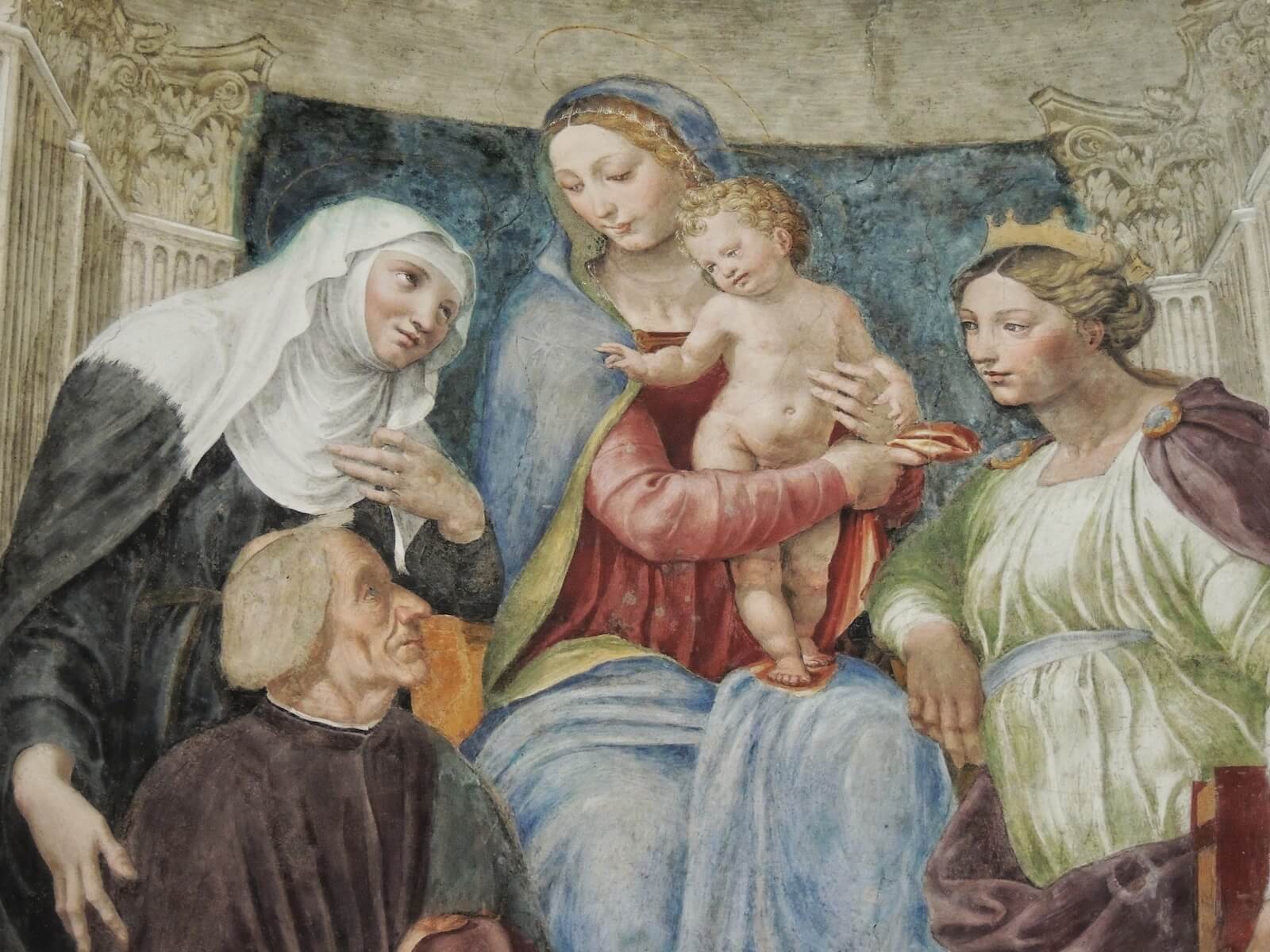This artwork, presumably centuries old and depicting a religious scene, portrays the biblical Mary and baby Jesus surrounded by several figures. At the center, Mary is clothed in a traditional blue robe with a red dress underneath and a cloak around her head. She is gently holding the unclothed baby Jesus, whose curly hair rests against her arm as she modestly shields his private area. Both Mary and Jesus are gazing downwards towards a monk situated at the bottom of the painting on the left side. The monk, identified by his shaved head, is looking adoringly upwards at the baby Jesus. Above the monk, slightly to the left, a nun dressed in a dark cloak with a white head wrap is also looking upwards in reverence towards Mary and the child. On the right side of the painting, a woman wearing a gold crown and adorned in a green flowing dress with a burgundy cloak gazes in their direction. The setting appears to be a grand hall, indicated by ornate carvings and marble decorative columns in the background, lending an air of solemnity and grandeur to this religious tableau.